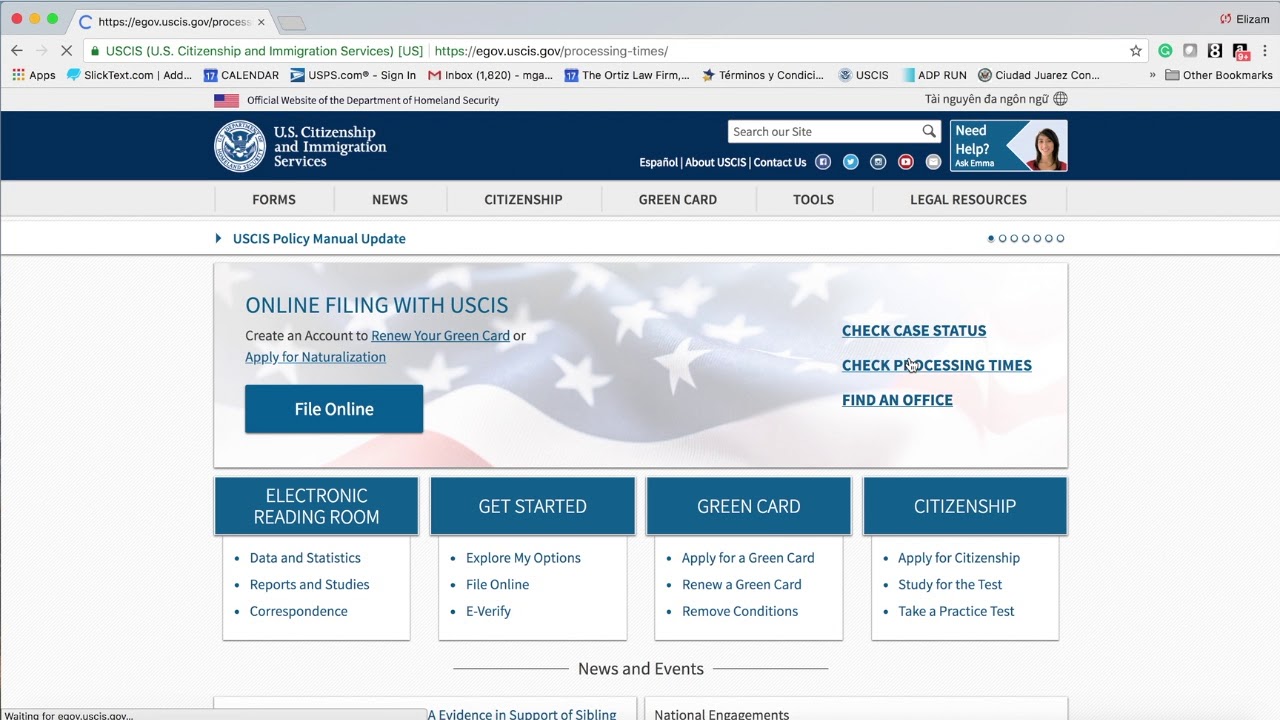This image displays a computer monitor showcasing a website related to immigration, specifically the U.S. Citizenship and Immigration Services (USCIS) site. The browser window is framed in a typical gray, commonly seen in Windows operating systems. In the top left corner, there are red, yellow, and green dots, indicating a likely use of Google Chrome. The URL visible in the address bar starts with "egov.uscis.gov/PROCES." 

The main text in the white bar reads "U.S. Citizenship and Immigration Services." Above this, a blue banner spans the width of the screen, displaying "U.S. Citizenship and Immigration Services | Search our Site" along with a prominent search box and a "Need Help" section to the right.

Directly below this banner, there is a gray navigation menu with the labels: "Forms," "News," "Citizenship," "Green Card," "Tools," and "Legal Resources." An eye-catching image beneath the menu promotes online services, stating: "Online filing with USCIS: Create an account, renew your Green Card, or apply for naturalization." Below this promotional section is a blue button with white text saying "File Online."

At the bottom of the page, there is a division into four square sections, each with a dark blue background and white lettering. From left to right, the sections are labeled: "Electronic Reading Room," "Get Started," "Green Card," and "Citizenship."

Additional links are present near the bottom, including one for "News and Events" and another partially visible link regarding "Evidence in Support of Sibling." To the right side, there is a link titled "National Engagements."

The user's bookmarked toolbar is also visible across the top edge of the gray area, displaying various bookmarked items. 

This detailed and organized layout effectively highlights the USCIS's online tools and resources for users navigating immigration processes.